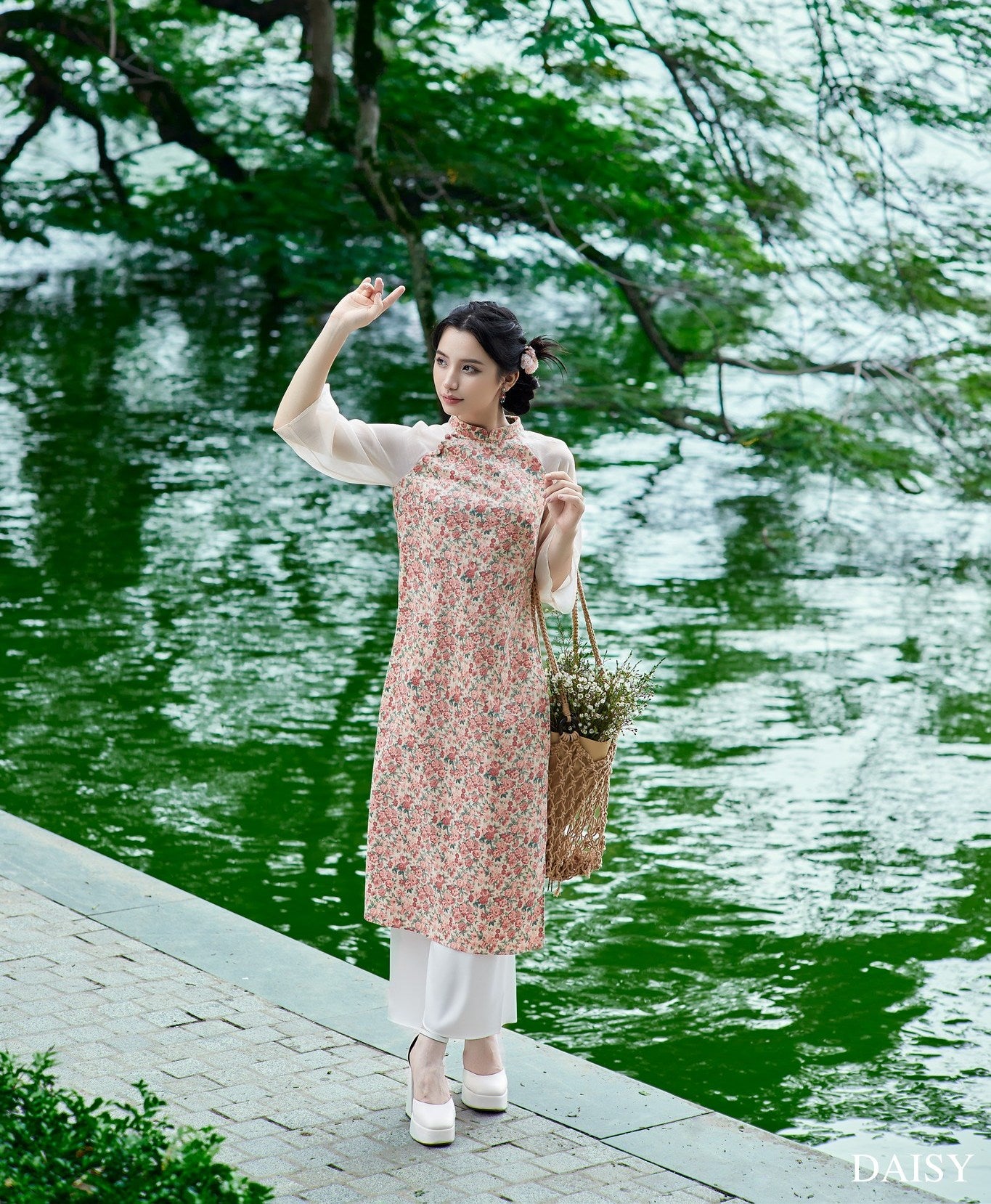The image is a color photograph capturing an East Asian woman, possibly a model, posing elegantly in a picturesque park setting by a green body of water. She is dressed in a layered ensemble featuring a knee-length floral dress with shades of pink and green over a longer, white underdress that reaches her ankles. The dress includes distinctive diaphanous white gauze sleeves that extend just past her elbows. She is wearing white high-heeled platform shoes. Her dark hair is tied back, adorned with flowers. In her left arm, she carries a loosely woven beige basket filled with flowers and greenery. The backdrop consists of a dark gray paved area she stands on, with overhanging tree branches reflecting green and white hues onto the water. To her left is a green hedge seen in the lower-left corner of the frame, adding to the serene, natural ambiance of the scene.